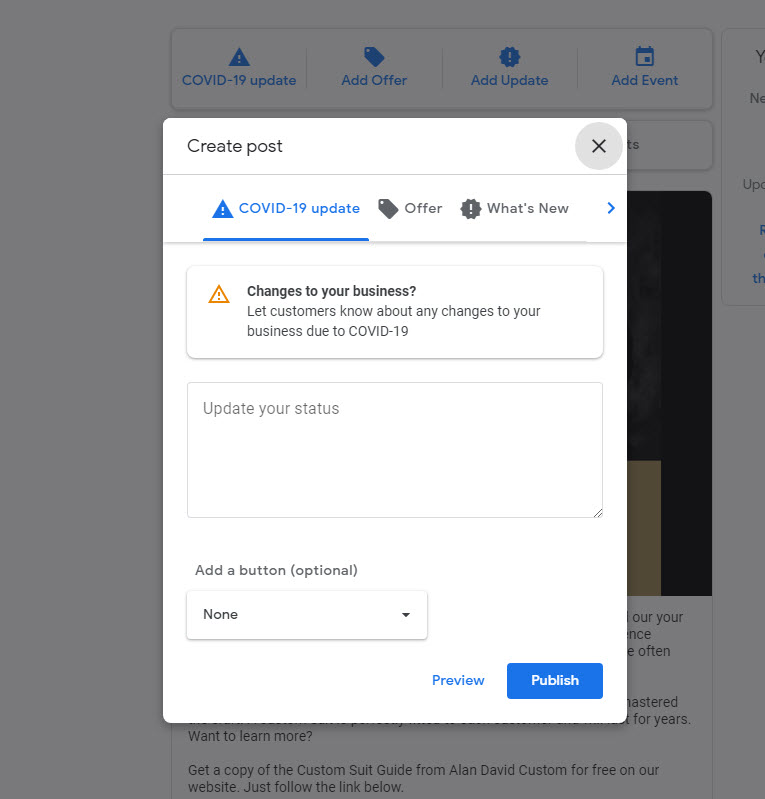This is an image of a website interface displaying a pop-up notification titled "COVID-19 Update." The notification, positioned on top of the webpage, obscures part of an underlying image that has a black background. The pop-up features various highlighted options, all in blue, including "Add Offer," "Add Update," and "Add Event." 

In the top-left corner of the pop-up, a large underlined blue text reads "Create Post," accompanied by an X enclosed in a gray circle on the top-right corner for closing the window. 

Within the pop-up, the text "COVID-19 Update" appears prominently underlined and flanked by a blue square containing an exclamation point. Below this, the word "Offer" is featured next to a ticket icon, followed by "What's New" next to a settings-type icon with a blue arrow pointing to the right.

Centrally located in the pop-up, the heading "Changes to Your Business" is marked by a red triangle with an exclamation point. This section encourages business owners to inform customers of any modifications due to COVID-19, featuring the text: "Let customers know about any changes to your business due to COVID-19."

The following section titled "Update Your Status" includes a large text field for custom input. Beneath this, there's an option labeled "Add a Button (Optional)" with the current selection set to "None" and a drop-down arrow for additional choices.

At the bottom of the pop-up, there are buttons for "Preview" and "Publish." The "Preview" button is highlighted in blue, while "Publish" is displayed in a darker blue box with white text.